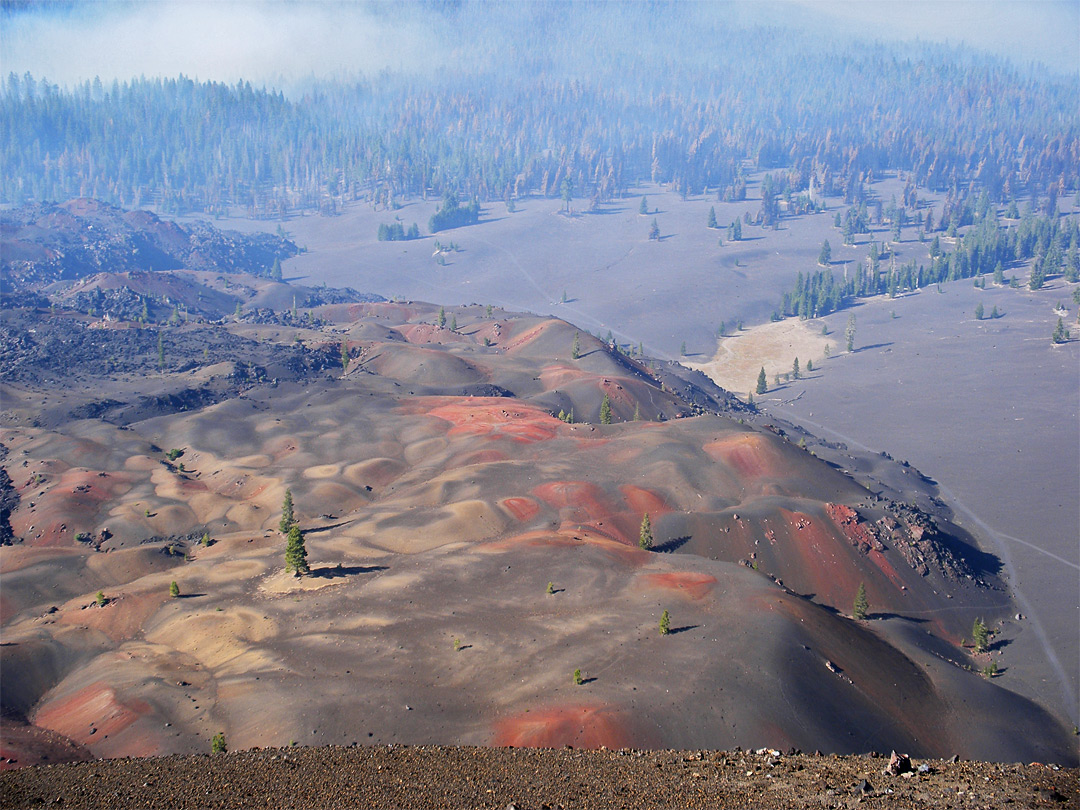The image captures a breathtaking bird's eye view of a mountainous and forested landscape, likely taken from the top of a mountain or a high vantage point. The foreground features rolling hills in shades of brown, red, and tan, with sparse green evergreens dotting the terrain. These hills appear almost clay-like and smooth to the touch. Descending from the hills, the landscape flattens into stretches of dark brown land interspersed with sandy patches, forming what seems like natural washes. A striking contrast unfolds in the distance where a dense forest of evergreen trees emerges, shrouded in thick white fog or clouds. The lush green of the forest starkly opposes the barren, almost desert-like terrain of the hills, creating a dramatic and visually captivating scene.